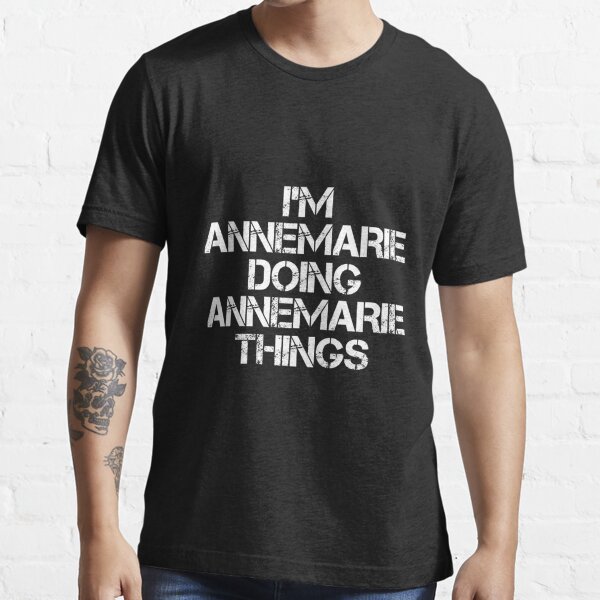The image depicts the midsection of a man standing against a white-painted brick wall. His face is not visible, as the shot is cropped from his neck to just below his waist. He is wearing a slightly long black t-shirt adorned with distressed white lettering that reads, "I'm Anne-Marie doing Anne-Marie things." The man is dressed in blue jeans. On his right arm, there is a black and white tattoo of a skull with a large rose and several leaves on top of the skull. Slightly lower on his inner arm, a partially visible tattoo appears to be the face of a large predatory cat, though the details are unclear. The image showcases him modeling the shirt, emphasizing his tattoos and attire.